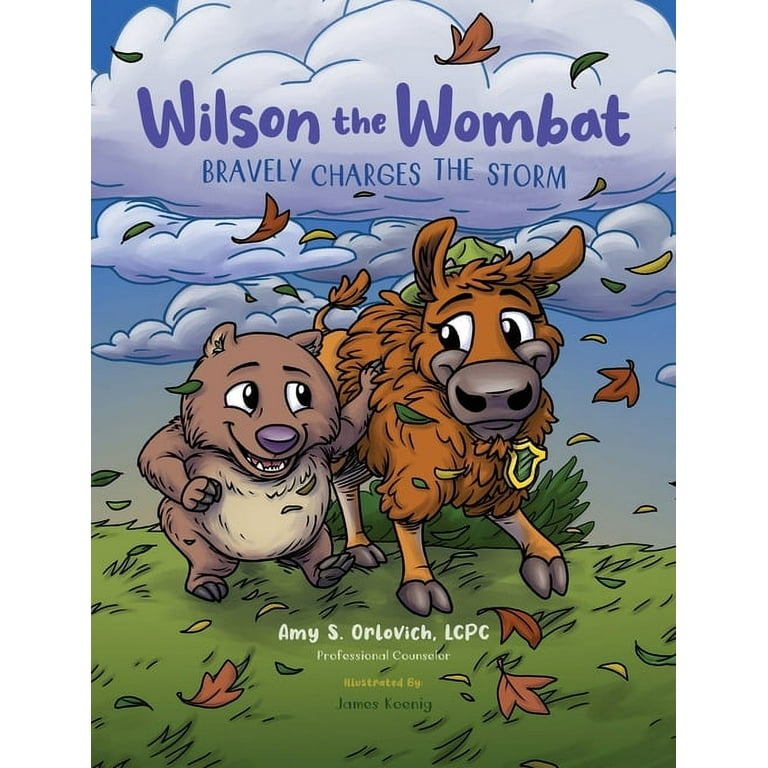This is an image of the front cover of a children's book titled, "Wilson the Wombat Bravely Charges the Storm," authored by Amy S. Orlovick, LCPC, and illustrated by James Koenig. The cheerful and cartoonish artwork features two characters: Wilson, a wombat, and his friend, a cow. The cow, colored in bright brown, wears a green ranger hat with a badge, while Wilson the wombat is accessory-free but exhibits a friendly demeanor as he paces alongside the cow. The cover portrays a very windy, cloudy day with leaves and grass blowing in the wind, suggesting an adventurous setting. Both characters are smiling at each other, exuding a sense of camaraderie and mutual encouragement despite the stormy weather.